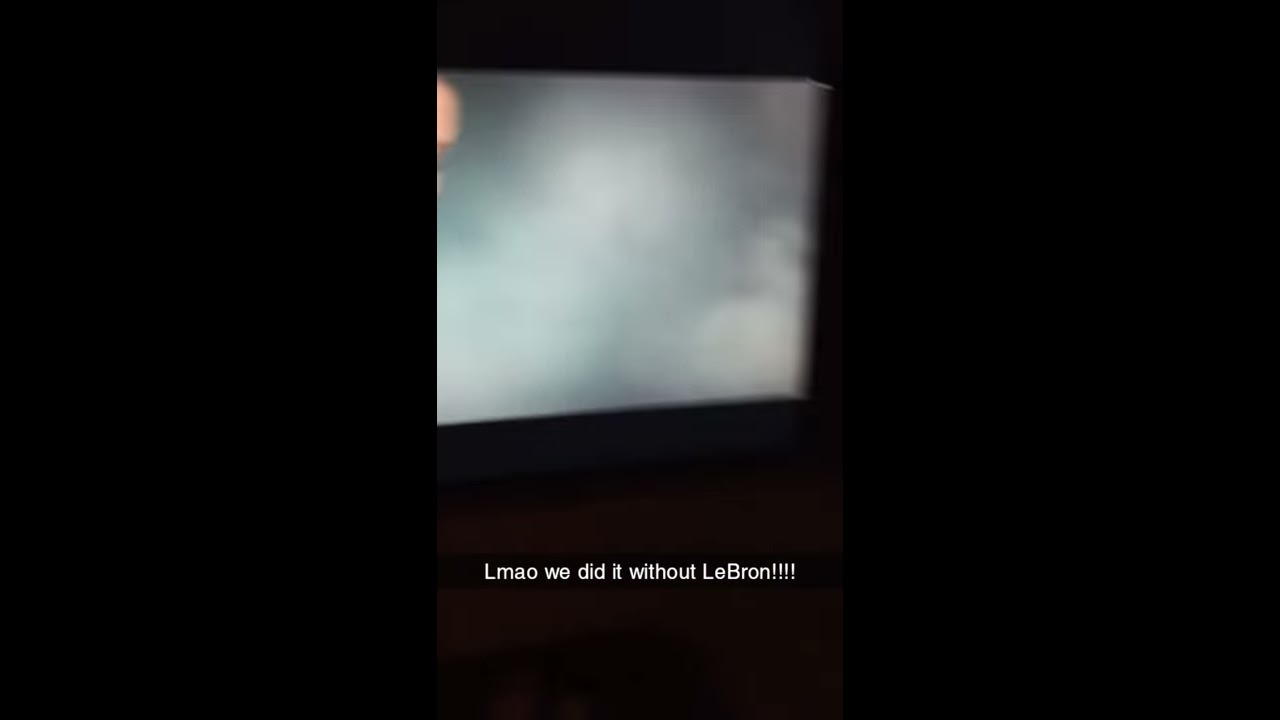The image depicts a predominantly dark scene with a hazy and out-of-focus television screen positioned centrally. The TV appears to be placed on a stand or a shelf, which slightly lights up the surrounding area with a faint grayish-blue glow that contrasts the otherwise dim room. Smoke or a cloudy effect is visible on the screen, adding to the blurry and soft, airbrush-like quality of the image. The text displayed at the bottom of the screen stands out clearly despite the overall lack of focus: "LMAO, we did it without LeBron!", emphasized with multiple exclamation points. This suggests that the TV is broadcasting a basketball-related video, possibly a celebratory clip from a social media platform like TikTok.